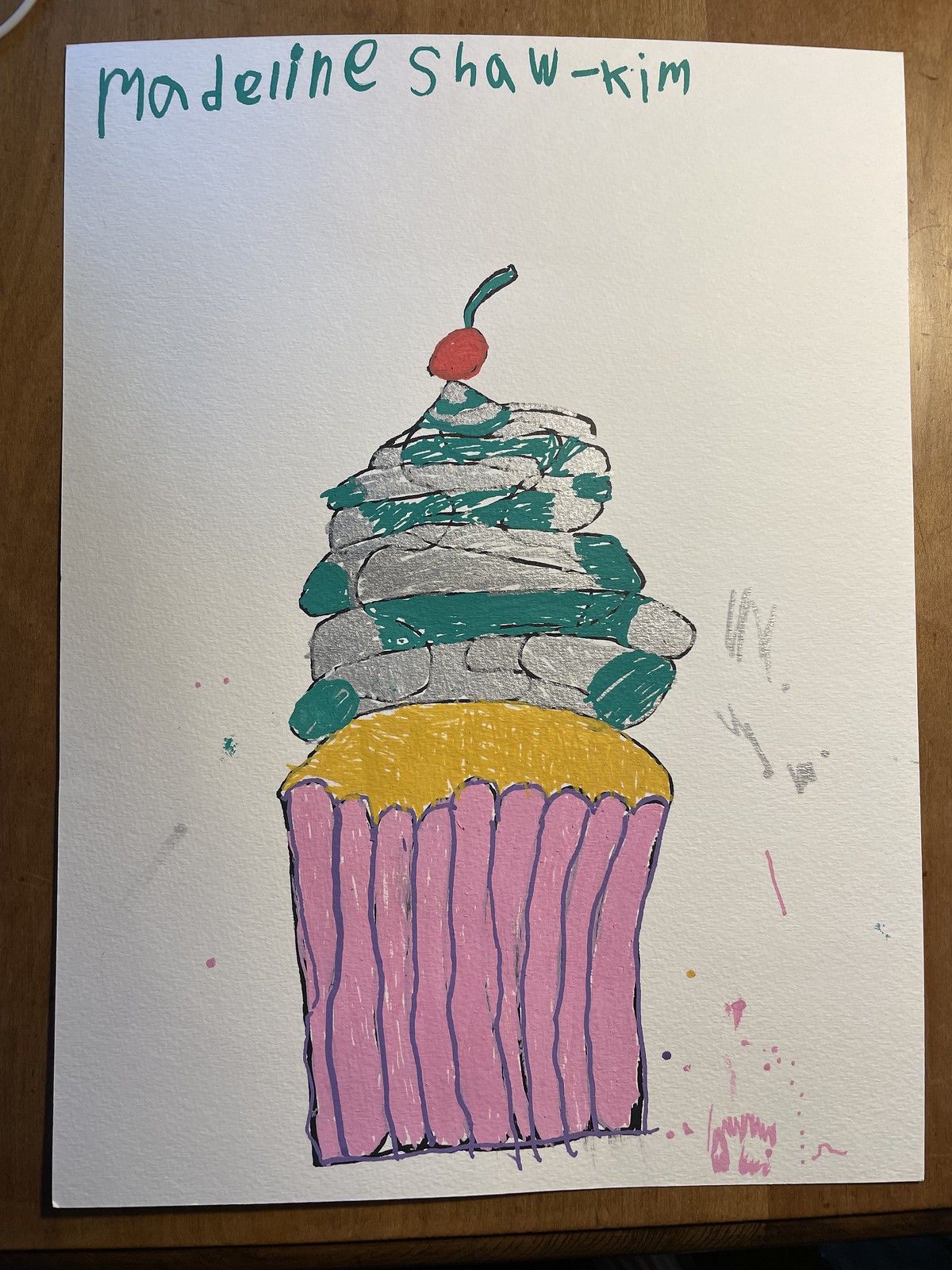This image depicts a child's drawing of a tall, whimsical cupcake created by Madeleine Shaw Kim, as indicated by the name written at the top. The cupcake features a vividly pink outer wrapper and a golden-hued sponge base. Towering above, a voluminous swirl of silver and teal cream or ice cream is artistically layered, crowned with a small, bright red cherry on top. The drawing is adorned with child-like pen markings along the sides, adding to its charming, hand-drawn quality.